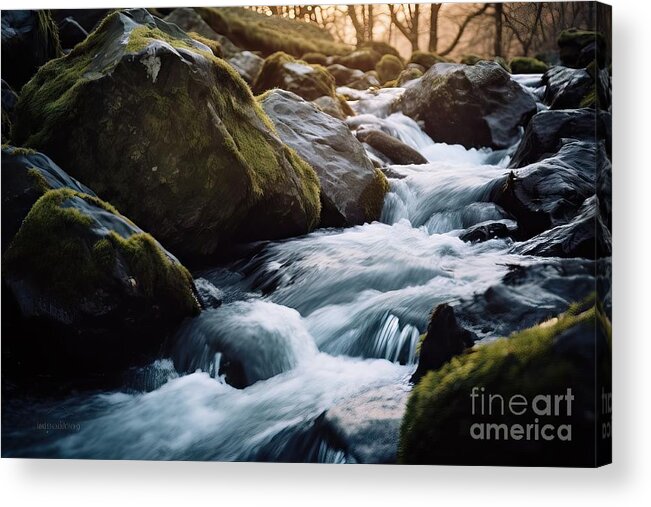This image, an art print on a three-dimensional canvas by Fine Art America, depicts a realistic and vibrant scene of a rushing white-water stream cascading down a series of craggy, jagged rocks. The powerful water, predominantly white and frothy, creates a dynamic sense of movement as it flows over the rocky terrain. The large gray boulders flanking the stream are sporadically covered in soft green moss, with the left side being more densely covered than the right. In the background, through the bare branches of several leafless trees, a golden, pinkish-orange light from either a rising or setting sun adds a warm, ethereal glow to the scene, hinting at an autumn or winter setting. The overall composition is further enhanced by the subtle gray text in the lower right corner, "Fine Art America," with the "Art" in slightly bolder font, marking the piece as a fine art creation.